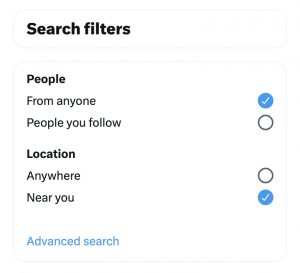The image shows a digital interface, likely from a computer or phone, with a white background. At the top left, there's a rectangular box outlined in light gray that contains black text reading "Search Filters." Below this, there's a square outlined in light gray with the heading "People" in the upper left corner. It offers two filtering options: "From Anyone" and "People You Follow," each with a corresponding circle on the right. The circle next to "From Anyone" is checked.

Further down is a section labeled "Location" in black text. This section provides two choices: "Anywhere" and "Near You," each with a bubble to their right. The bubble next to "Near You" is selected, indicated by a blue circle with a white check mark inside.

At the bottom left of the interface, "Advanced Search" is written in light blue text, suggesting more detailed filtering options. The user's current filters include "From Anyone" under the People section and "Near You" under the Location section, indicating they are refining their search criteria based on these preferences.